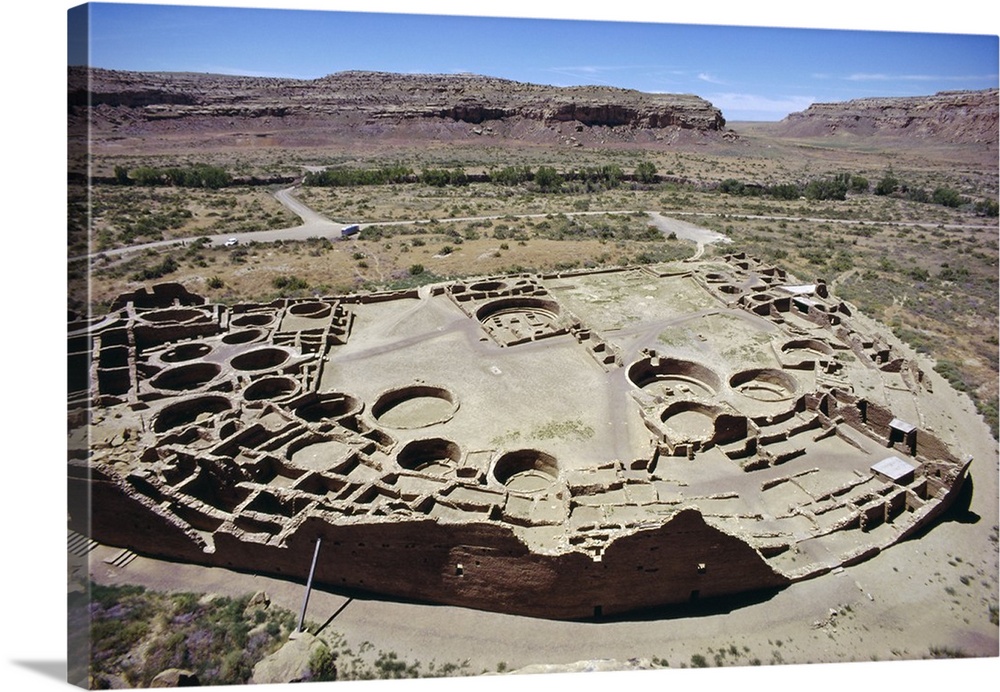This is an overhead photograph depicting the ruins of what appears to be an ancient Indian settlement, possibly located in the desert regions of South Dakota or Navajo territory. The focal point of the image is a large circular structure, resembling an amphitheater, made of white clay or stone. Surrounding this open area are remnants of adobe walls that have mostly crumbled away, leaving a tan, mud-like appearance. The setting is distinctly desert-like, with sparse scrubby green vegetation and predominantly brown terrain. In the background, majestic mesas and a rocky mountain range are visible under a clear blue sky with a few clouds. A singular road leads to this settlement and extends into the distance, giving a sense of isolation and desolation. There is no visible text or artist's trademark on the canvas, and the photo captures the harsh, arid landscape with remarkable clarity and detail.